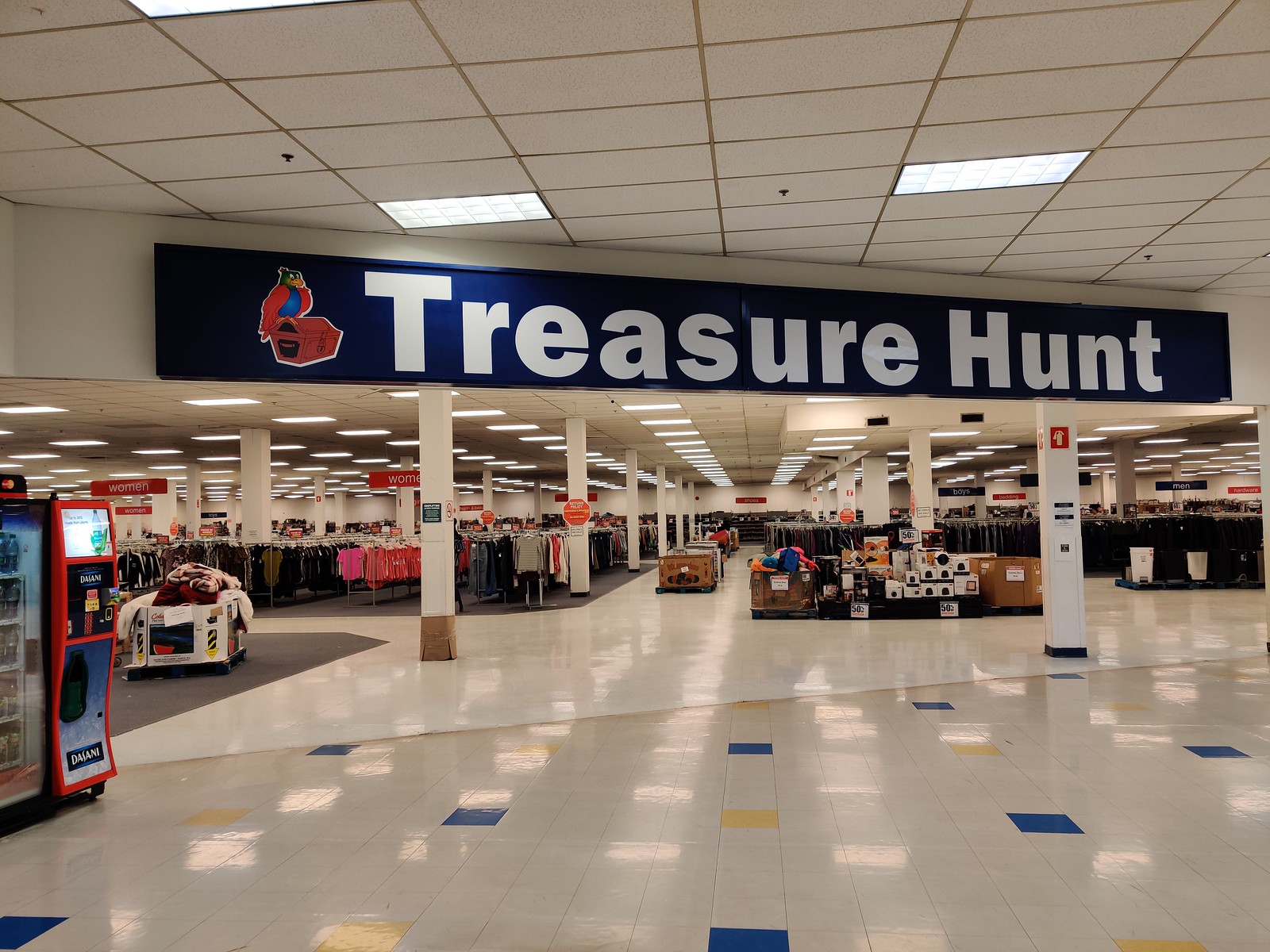This image captures the interior of a spacious retail store named "Treasure Hunt," prominently indicated by a large sign with white letters on a dark blue background. The store features a striking floor design, with white linoleum tiles interspersed with dark blue and yellow squares. Multiple aisles showcase a variety of merchandise, including clothing and other goods. On the left side, there is a table displaying additional items. Further to the left, a machine—potentially a vending machine or an arcade game with a red trim—catches the eye. The store extends far into the background, revealing its large size, characterized by a drop ceiling and illuminated by fluorescent lights. The space is further defined by white pillars distributed throughout, providing structural support.